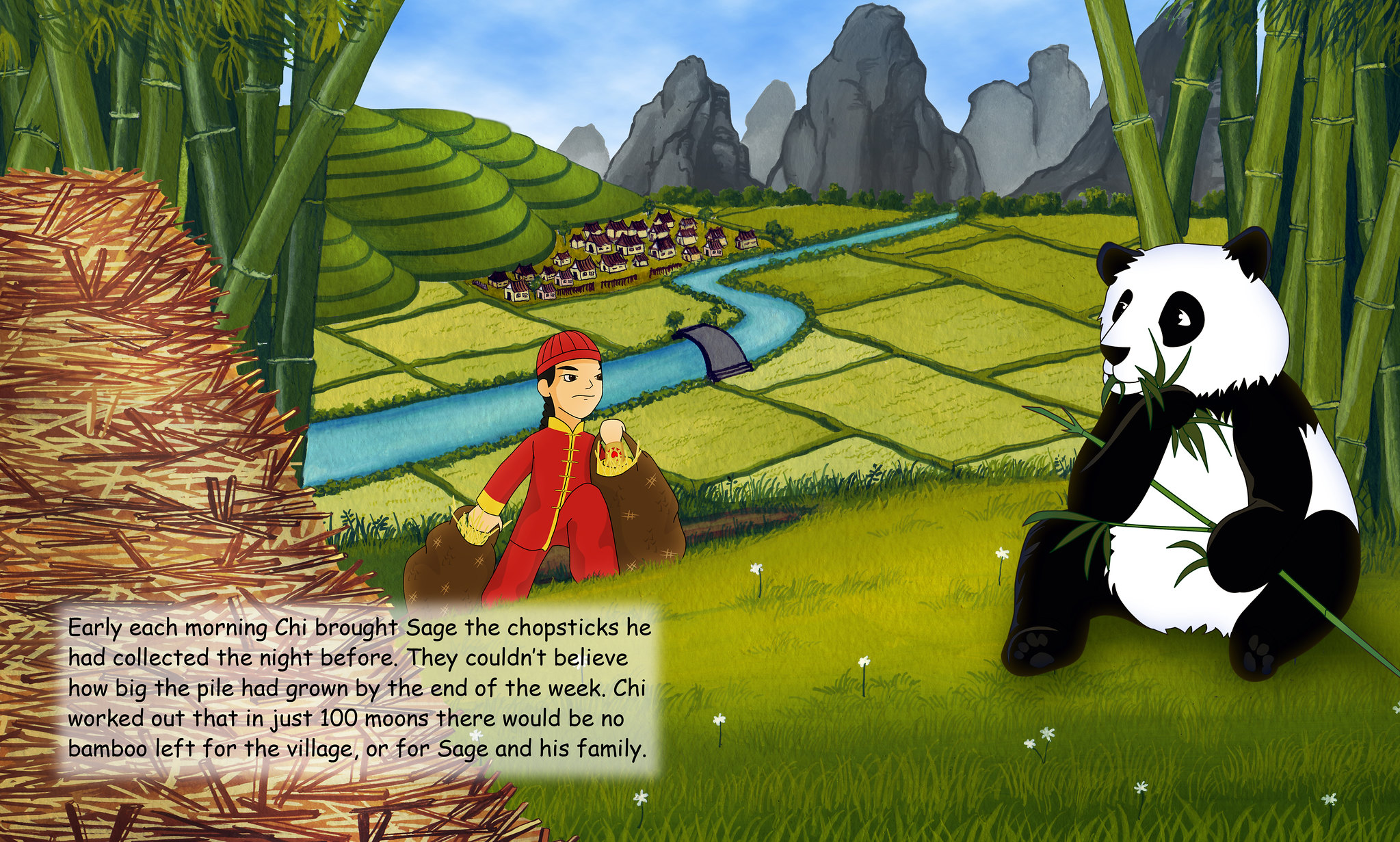In this vibrant and detailed illustration from a Chinese children's book, a small boy named Qi, who appears to be around 10 years old, is the central focus. He wears a red and gold traditional outfit and is shown ascending a hill, carrying two large brown bags full of plants. The background reveals lush rice paddies transitioning into a quaint town nestled in the shadows of towering grey stone mountains. To the right of the scene, a large, portly panda sits comfortably among the bamboo, munching on leaves and seemingly staring at Qi. The lush setting is dotted with dandelions, adding charm to the picturesque landscape. Text on the image reads: "Early each morning, Qi brought Sage the chopsticks he had collected the night before. They couldn't believe how big the pile had grown by the end of the week. Qi worked out that in just 100 moons, there would be no bamboo left for the village or for Sage and his family." The image combines elements of nature, tradition, and storytelling to create a rich, immersive scene.